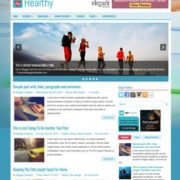The image depicts the homepage of a website called "Healthy," which prominently features a pink heart logo set against a blue background. The word "Healthy" is stylishly presented in teal. The website includes a navigation bar with multiple clickable tabs, each labeled in blue font. The homepage dynamically cycles through various health-related articles.

Currently, the featured article showcases an outdoor scene with five individuals, possibly on a beach or hiking in nature, under a sky filled with clouds. Additional articles displayed on the homepage include one with an image of a yellow taxi cab, and another featuring a person inserting a small credit card or wallet at a computer keyboard.

The website design incorporates social media icons, enabling users to follow "Healthy" across different platforms. There are sections for related articles and other informative content, all aimed at delivering health-focused information. The overall color scheme of the site is predominantly blue, complemented by white and various text styles, creating a cohesive and inviting aesthetic.